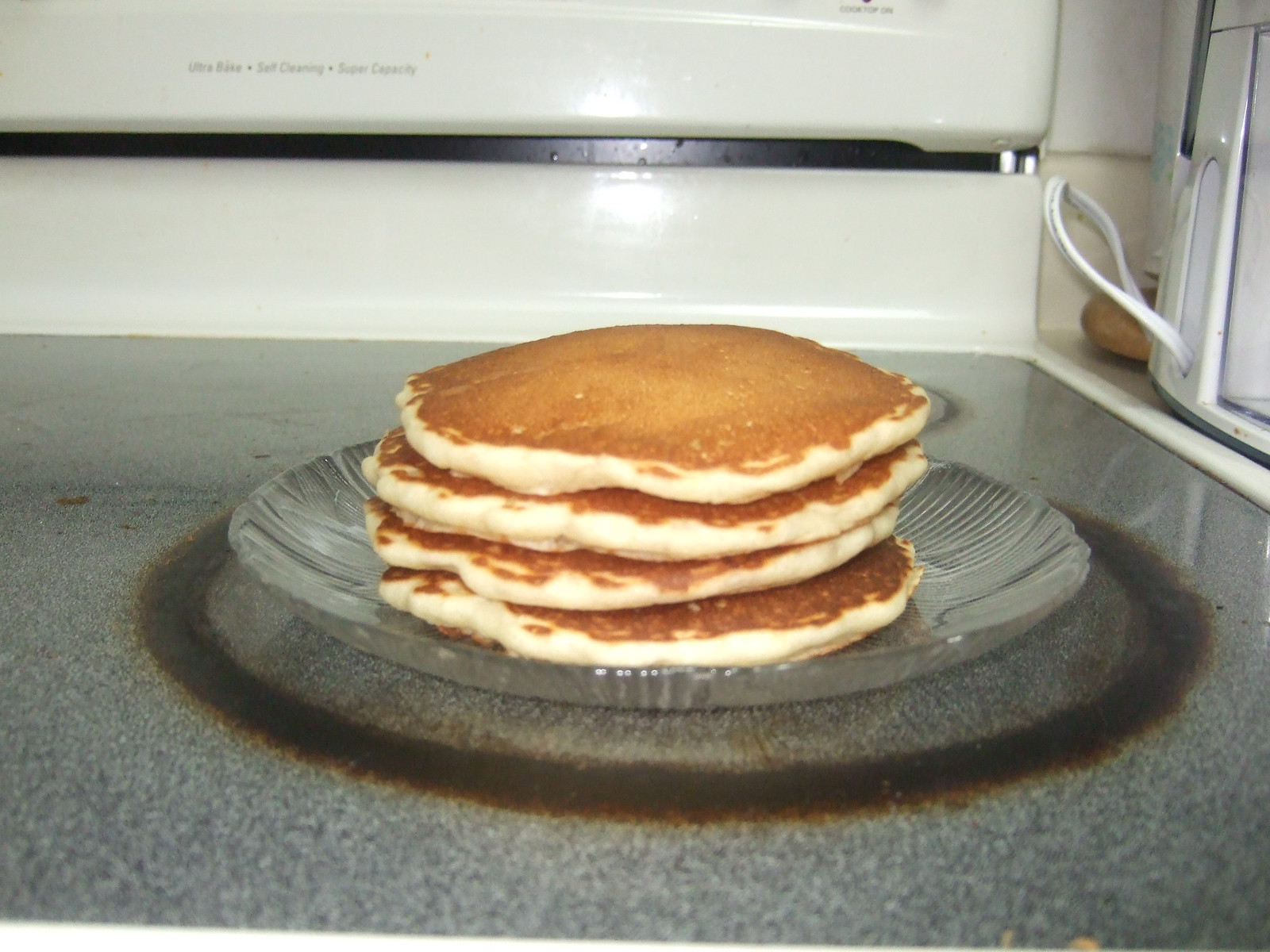The photograph captures a detailed, close-up view of an off-white induction stovetop with a smooth, gray-speckled glass surface. Centrally positioned is a transparent glass plate, resembling a shallow bowl, bearing a stack of four evenly browned pancakes. The pancakes, approximately six inches in diameter, are plain and precisely cooked, without any syrup. Surrounding the burner, a conspicuous brown burn mark indicates previous overuse. In the background, partially visible, there’s a white coffee maker situated to the right side of the image. The overall aesthetic highlights the food against the clean, modern lines of the kitchen appliance.